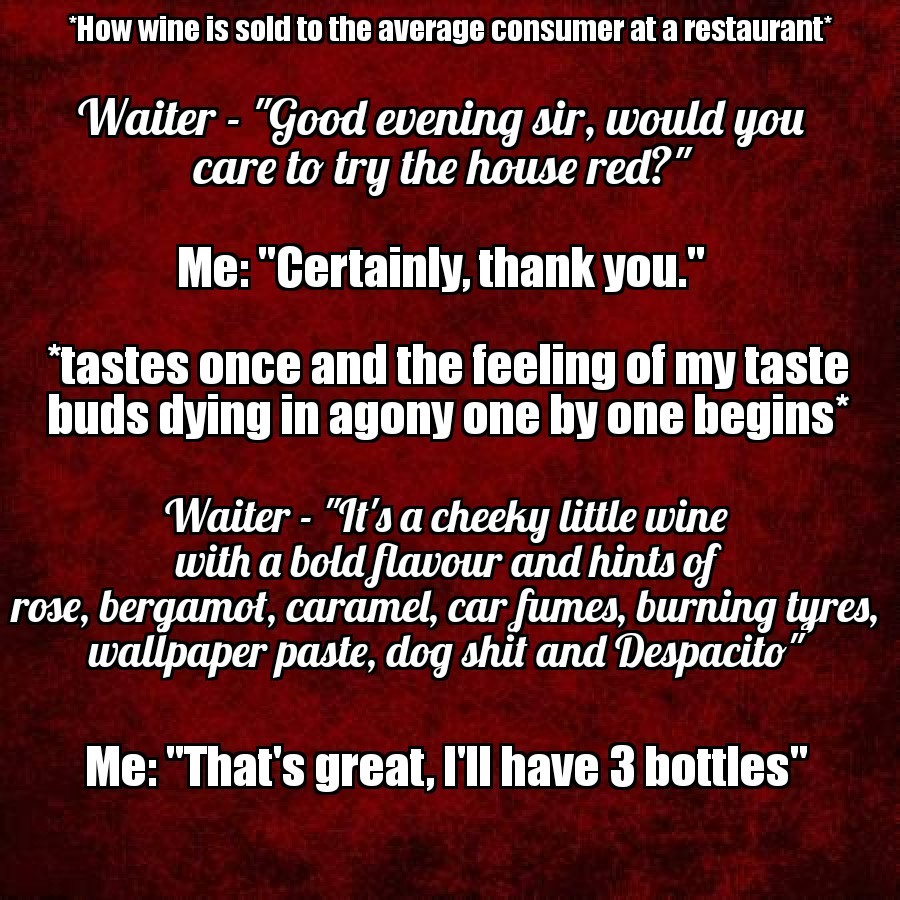The image is a humorous textual meme with a burgundy background featuring fancy gradients and red smoke effects. The text is entirely in white, with some parts outlined in black. The title, "How Wine is Sold to the Average Consumer at a Restaurant," is slightly smaller than the rest and serves as the introduction to a satirical dialogue. 

The text is formatted as a conversation where a waiter says, "Good evening sir, would you care to try the house red?" to which the customer replies, "Certainly, thank you." The next line humorously describes the customer's reaction: "Taste once and the feeling of my taste buds dying in agony one by one begins." The waiter continues with an exaggeratedly bad wine description: "It's a cheeky little wine with a bold flavor and hints of rose, bergamot, caramel, car fumes, burning tires, wallpaper paste, dog shit, and despacito." The customer comically concludes with, "That's great, I'll have three bottles."

The waiter's text is italicized to distinguish it from the block text of the customer, adding to the comedic effect. This satirical piece pokes fun at the pretentiousness surrounding wine culture in restaurants.